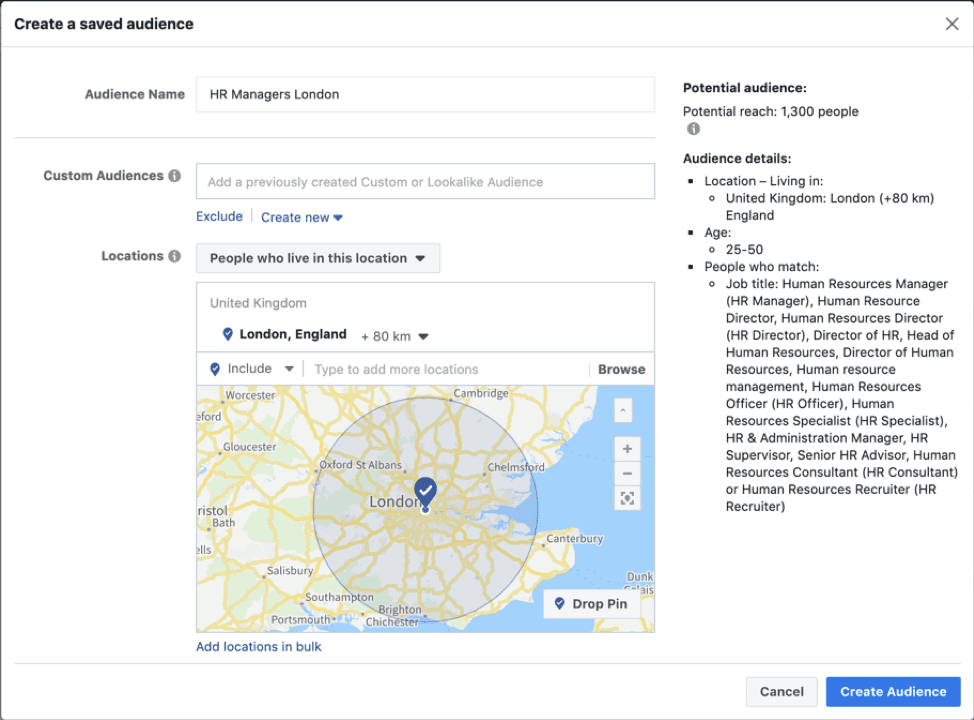Here's a detailed descriptive caption for the provided image:

---

This screenshot is from a job listing or audience targeting site, capturing the interface of creating a saved audience for targeted job advertisements. 

### Key Elements:

- **Top Section:**
  - **Header:** "Create a Saved Audience" is prominently displayed in bold in the top-left corner.
  - **Close Button:** An "X" symbol in the top-right corner allows users to close the window.

- **Audience Naming:**
  - **Input Field:** A blank space to name the audience, currently filled with "HR managers London."

- **Custom Audiences:**
  - **Options:** A section titled "Custom Audiences" with a prompt to "Add or previously created custom or lookalike audience."
  - **Exclusion Settings:** Includes an "Exclude" option and a "Create new" dropdown arrow.

- **Location Settings:**
  - **Dropdown Menu:** Set to "People who live in this location."
  - **Map Display:** Shows a detailed map of the United Kingdom, focusing on London and its surrounding area within an 80-kilometer radius.
  - **Location Management:** Features options to include or add more locations, facilitated by a search bar or browsing tool.
  - **Bulk Addition:** A button is available to "Add locations in bulk."

- **Right Side:**
  - **Audience Data:** A completely white background displaying potential reach and detailed audience information.
  - **Potential Reach:** Indicates a potential audience size of 1,300 people.
  - **Audience Details:**
    - **Location:** Living in the United Kingdom, London + 80 kilometers.
    - **Age Range:** 25 to 50 years old.
    - **Job Titles:** Specifies various Human Resources-related titles such as HR Manager, HR Director, Director of HR, and Head of HR.

- **Action Buttons:**
  - **Cancel:** Option to cancel the creation process.
  - **Create Audience:** A prominent blue button to finalize and create the audience.

---

This detailed caption captures the essence of the screenshot, describing each element and its function to provide a clearer understanding of the interface.